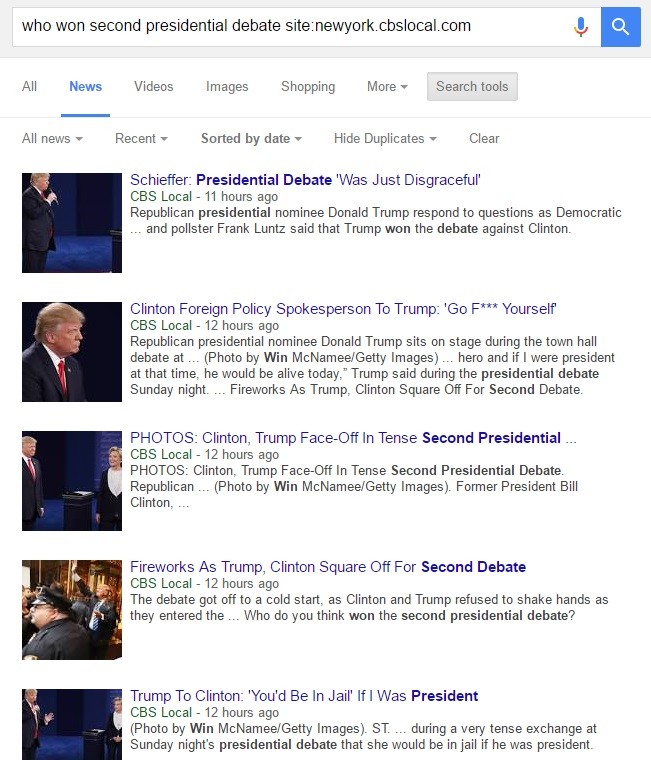A screenshot captures the results of a search query typed into a browser, specifically "who won second presidential debate site: NewYork.cbslocal.com." At the top of the image, there is a search bar with some white space to its right, followed by a microphone icon and a blue search button featuring a magnifying glass. Below the search bar, navigation options labeled "All," "News," "Videos," "Images," "Shopping," and "More" are displayed, along with a "Search tools" option. The "News" tab is selected, indicated by its blue outline and underline.

The search results reveal various articles related to the second presidential debate. Each article features a thumbnail image on the left and a text summary on the right. Many of the thumbnails depict Donald Trump, with a couple showing Hillary Clinton. The top article is titled, "Schiffer: Presidential Debate Was Just Disgraceful" from CBS Local, posted 11 hours ago. Another prominent headline reads, "Clinton Foreign Policy to Trump: Go F Yourself," accompanied by a description mentioning photos of Clinton and Trump facing off in a tense debate. Additional snippets and images further detail coverage of the event.